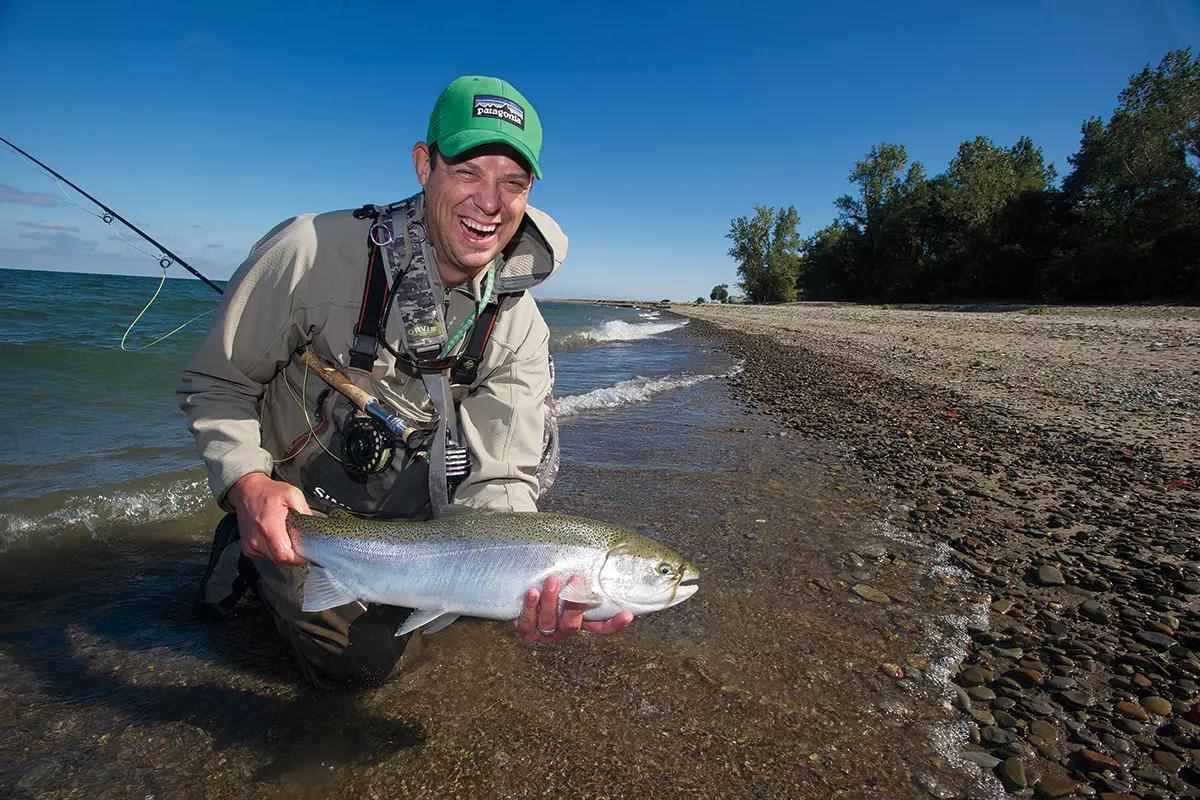In this close-up, color photograph, a jubilant fisherman kneels on a rocky beach, proudly displaying a large, silver-colored fish with two bottom fins in both hands. He wears a green baseball cap featuring a Patagonia logo and a broad, delighted smile on his face. His attire consists of a hooded gray, possibly white, jacket, long brown pants, and gray boots. The shoreline extends into the background, with rolling waves meeting the beach and a small wooded area to the right. His fishing rod is tucked securely under his right arm, pointing out of frame, completing the scene on this bright blue-sky day.